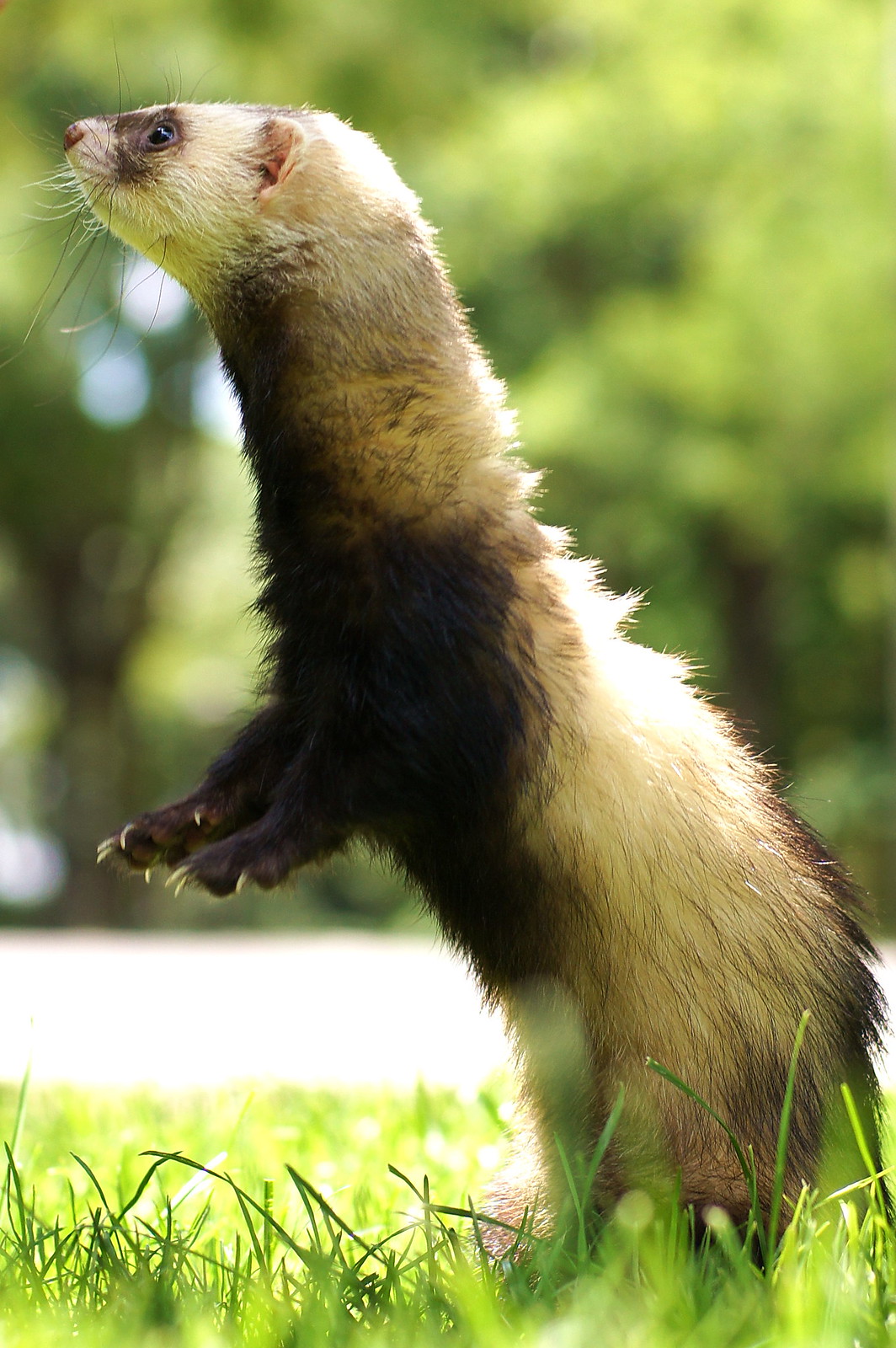This is a detailed digital photograph of a cute, fluffy ferret standing outside in a small field of tall green grass. The ferret, weighing approximately 10 to 15 pounds and measuring about one to two feet in length, is positioned on its hind legs with its forelegs raised. Its gaze is directed to the left of the image as it looks off into the distance at something intriguing. The ferret's fur is a combination of black, blackish-brown, and white. Its back is predominantly white, while its neck, belly, chest, and forearms are black. It also features distinct dark brown and black rings around its eyes and long black whiskers. Behind the ferret, the background is slightly blurry but reveals a roadway or path and some trees with sunlight filtering through, creating a serene outdoor atmosphere. The image is of high quality, clearly showcasing the ferret's fingernails, individual hair spikes, and the blades of grass around it.